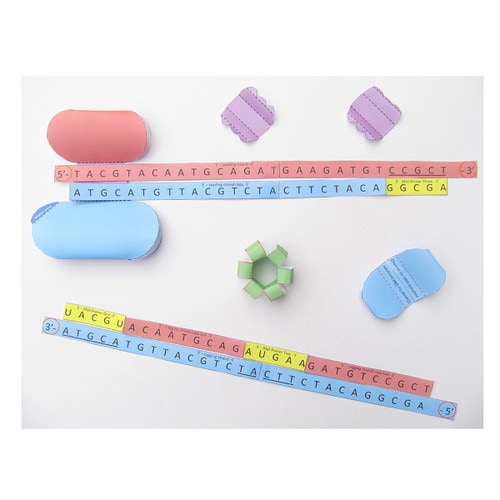The image features a detailed model for understanding DNA replication, staged against a plain white background. Central to the composition are rulers or strips that represent DNA strands, arranged horizontally. Near the top quarter, a pink strip with black letters (T, A, C, G) extends from the 5' to the 3' end, complemented by an underlying blue strip with corresponding letters following standard DNA base-pair rules—T pairs with A, and C pairs with G. Notably, the last five letters on this strip are highlighted in yellow.

A similar arrangement is present near the bottom quarter. This region starts with a yellow section and alternates between pink and blue sections, also following the complementary base-pairing rules with letters (A, T, G, C). Scattered around these key elements are various pastel-colored shapes resembling paper art, including a green flower-like form in the center and several butterfly-like shapes in blue and purple, adding decorative interest to the scientific model. To the left of the central floral shape is a blue pencil case-like object, while a pink elliptical object is located at the top and a similar colored item is at the bottom, echoing the rulers' color scheme. This meticulous assembly offers a vibrant yet precise representation of DNA replication mechanisms.